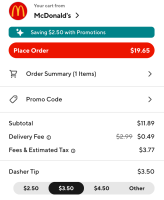This appears to be a detailed description of a screenshot from a mobile phone webpage showing a McDonald's order summary. The image comprises several elements that can be broken down as follows:

At the top of the screen, there is a McDonald's logo featuring the iconic yellow 'M' and the text "Your cart from McDonald's." Below the logo, a green horizontal bar contains white text that reads "Satan 250 with promotion," accompanied by a star icon on the left-hand side. 

Following this, a red rectangle with curved edges and white text indicates the "Place order 1965" button. In this section, black text on a white background reads "Order Summary" alongside a cart icon, and it mentions "1 item" with a right arrow next to it. There's also an option for entering a "Promo Code" marked by a little tag icon and another right arrow.

The cost breakdown begins with a subtotal of $11.89. The delivery fee initially listed as $2.99 has been reduced to $0.49, indicated by slashed-out text. Additionally, there’s an estimated tax of $3.77 with a small circular icon beside it. The 'Dasher tip' section shows a default selection of $3.50, but at the bottom, users can choose from various tip amounts: $2.50, $3.50 (highlighted in black), $4.50, or enter a custom amount.

This comprehensive view reflects the ordering process for a McDonald's delivery via a mobile app, showing the various steps and elements involved in finalizing the order.